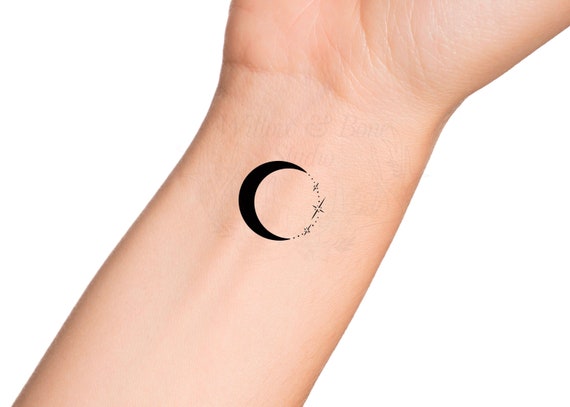This photograph is a close-up color image of a pale-skinned female's wrist and a portion of her forearm and hand. The focal point of the image is a tattoo, digitally superimposed onto her skin, consisting of a black crescent moon facing to the right. The moon sits prominently at the center of the wrist. Extending from the points of the crescent are a series of dots that form a circular pattern. This pattern features three stars: a larger star in the middle, flanked by two smaller stars. Above the moon, in faint, barely visible lettering, the words "Willow and Bone Studio" can be discerned. The background appears to be white or transparent, allowing the details of the tattoo and the paleness of the wrist to stand out. The orientation of the hand runs from the bottom left to the top right of the frame.